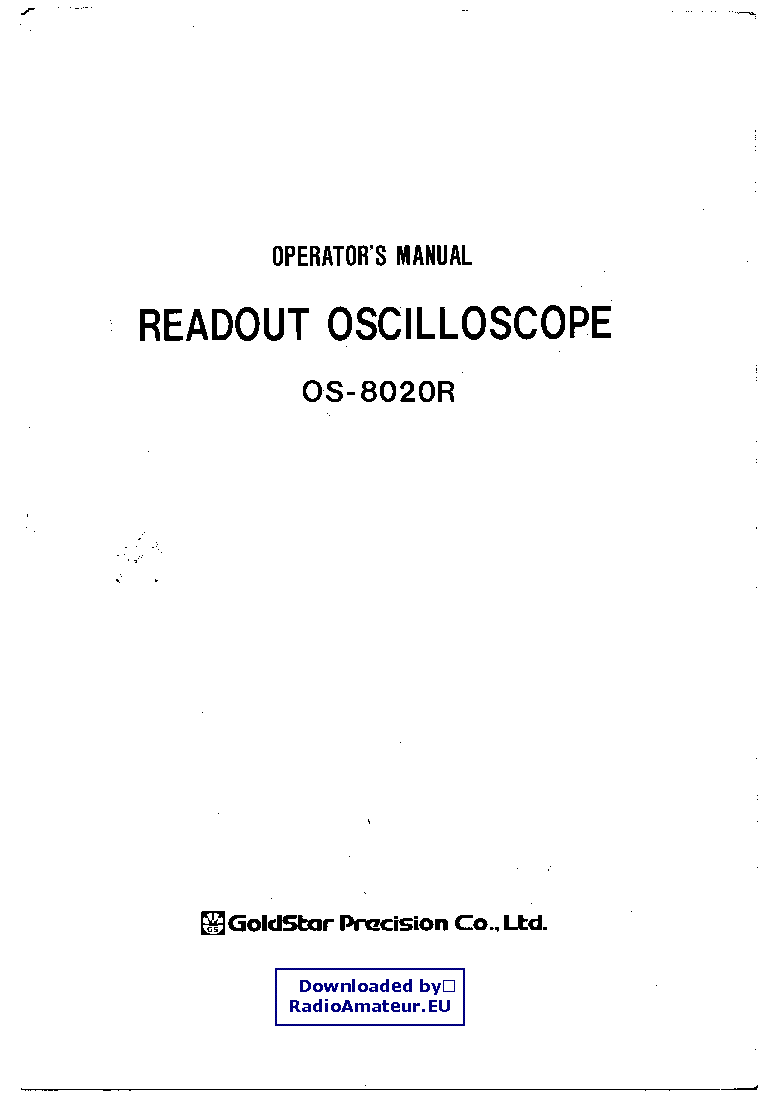The image is a scan of an "Operator's Manual" with an all-white background and black text. The title "Operator's Manual" is at the top in large capital letters. Below that, in even larger, bold capitals, it reads "Readout Oscilloscope." Further down, in smaller text, it says "OS-8020R." On the bottom left, there is a logo featuring a bowl containing a tool, an "L," and an inverted "L," with "GS" underneath and "Gold Star Precision Company, Ltd." to the right. At the bottom, enclosed in a blue-outlined rectangle, the text reads "Downloaded by RadioAmateur.eu."